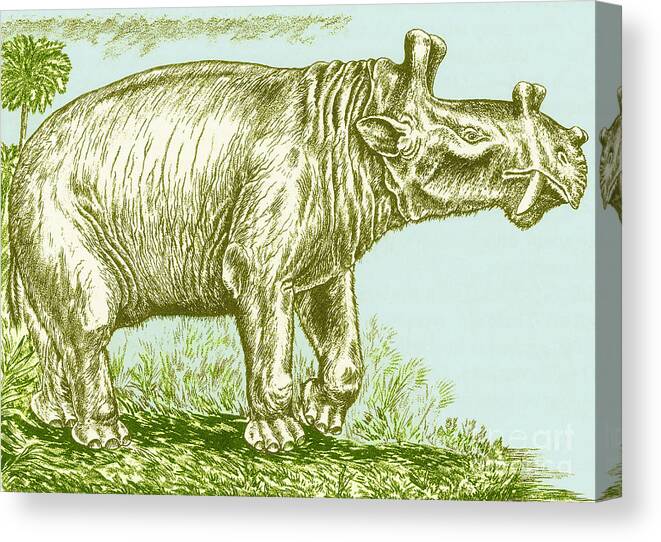The image depicts a detailed, sketched illustration of an indistinct creature that bears resemblance to both a hippopotamus and a rhinoceros, featuring characteristics such as elephant-like feet, a wrinkled neck, and downward-pointing tusks. The creature, drawn in various shades of green, appears to be walking on a grassy terrain that alternates between short and long patches. It is positioned centrally on a rectangular canvas with visible edges, the art medium resembling colored pencil. The background is a very light sky blue, interspersed with subtle green smudges, enhancing the vividness of the subject. To the left of the creature stands a green palm tree, adding a touch of tropical scenery to the composition. The animal is oriented facing right, with one foot raised as if in mid-stride, and a single eye and small horn-like features are discernible. The entire piece emanates a serene yet enigmatic aesthetic, making it a unique and captivating work of art.